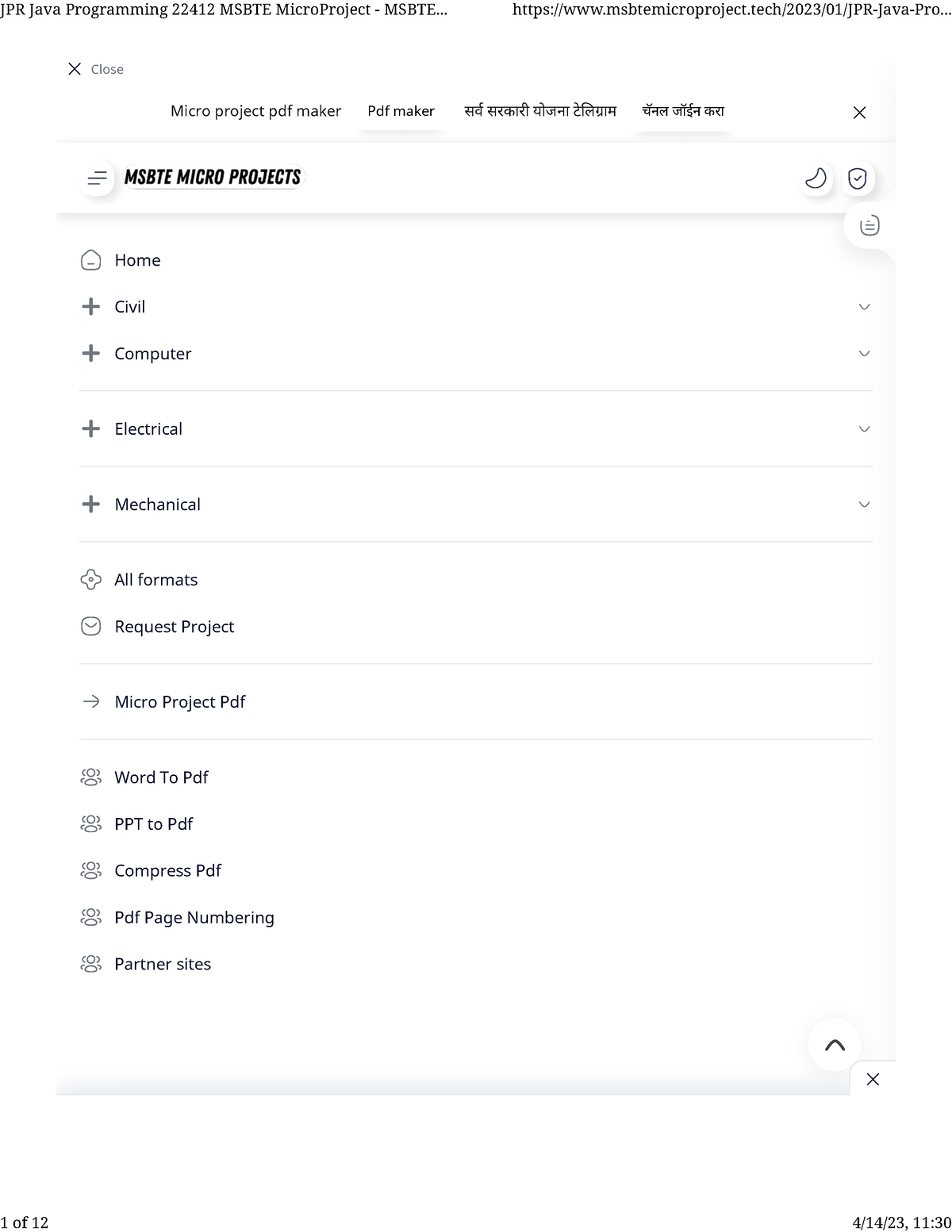This image is a screenshot from a website or app related to JPR Java Programming, appearing to originate from MSBTE Microprojects. In the top section, there are some numerical references and a hyperlink. The screenshot prominently features a pull-out or drop-down menu displaying various navigational options: Home, Civil, Computer, Electrical, Mechanical, All Formats, Request Project, Microproject, PDF, Word to PDF, PowerPoint to PDF, Compressed PDF, PDF Page Numbering, and Partner Sites. 

In the bottom right corner of the image, an upward-pointing arrow indicates an option to retract or minimize the menu. The top right corner hosts an X icon for closing the page and a moon symbol, likely for switching the website to dark mode. To the side of the moon symbol, a badge with a checkmark is visible, suggesting some form of verification or completion status. Additionally, there is a right-side pull-out menu, hinting at further expandable options.